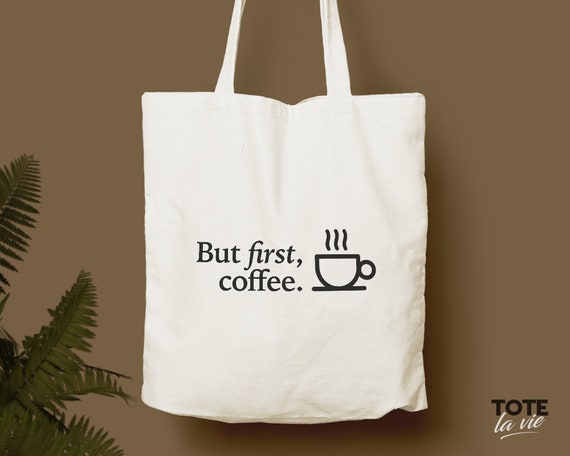This color image displays an off-white, linen canvas tote bag centered against a milk chocolate brown background. The tote bag, partially suspended from the top with the handle cut off, is adorned with the phrase "but first, coffee" in dark writing. Adjacent to the text is a simplistic, computer-generated drawing of a steaming coffee cup sitting on a saucer. Overlaying the bottom right corner, the words "TOTE LA VIE" appear, with 'TOTE' in black and 'LA VIE' in white, the latter underlined. A touch of greenery from what seems to be tall fern leaves peeks in from the bottom left of the image.